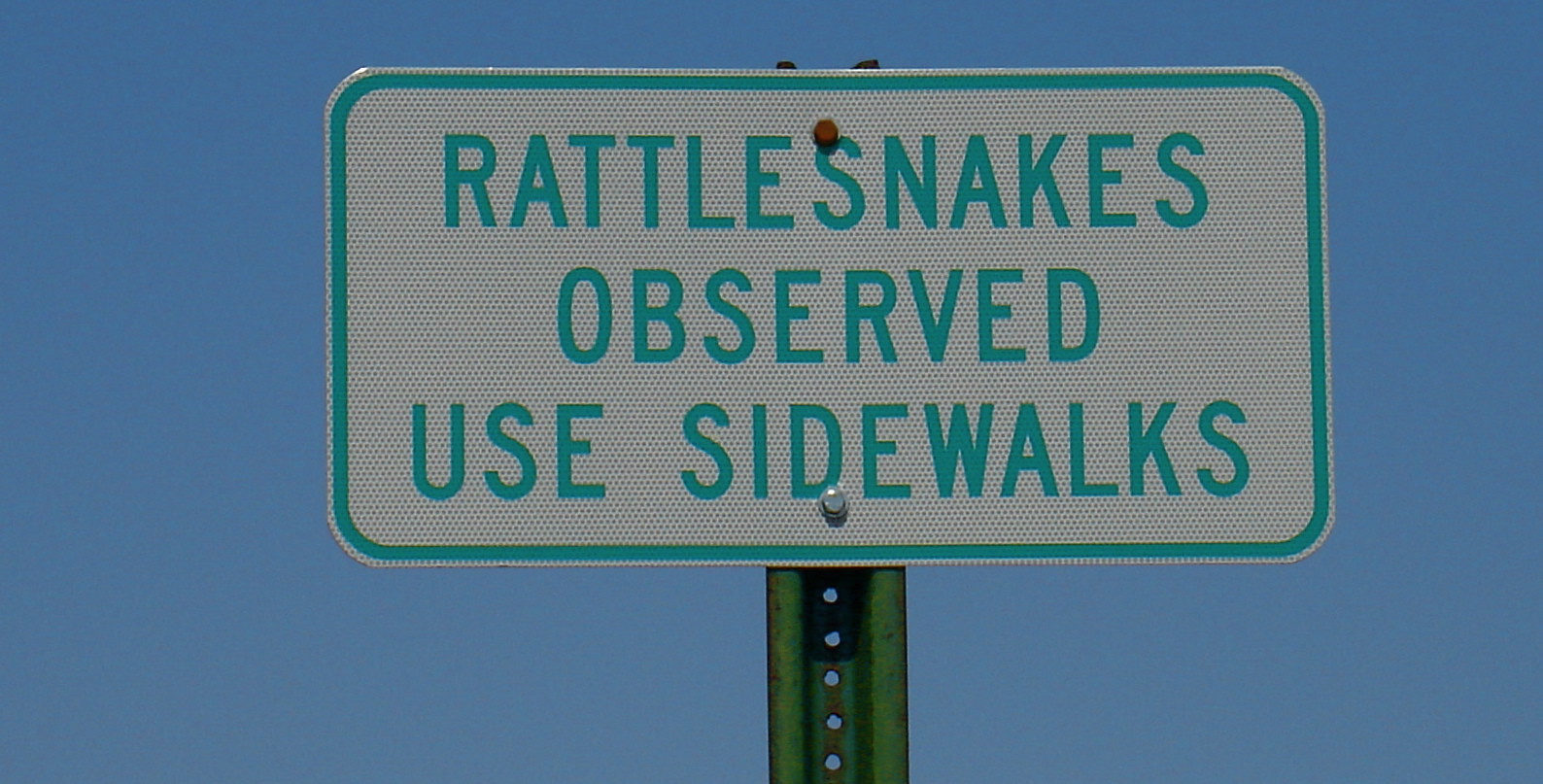This is a close-up color photograph taken outdoors, featuring a prominently displayed rectangular metal sign against a striking blue sky. The long side of the rectangle stretches horizontally from left to right. The sign itself is rimmed with a greenish aqua color and sports a white background with bold, greenish aqua lettering that reads: "RATTLESNAKES OBSERVED USE SIDEWALKS". The sign is securely fastened to an emerald green metal post with two visible bolts. The top of the post peeks out above the sign, then reappears below it, extending off the bottom of the image. This green post features multiple evenly spaced holes through its center, allowing glimpses of the clear blue sky to peek through. The sign's background also has subtle design elements, including faint squares of darkness, adding texture to its otherwise smooth white surface.